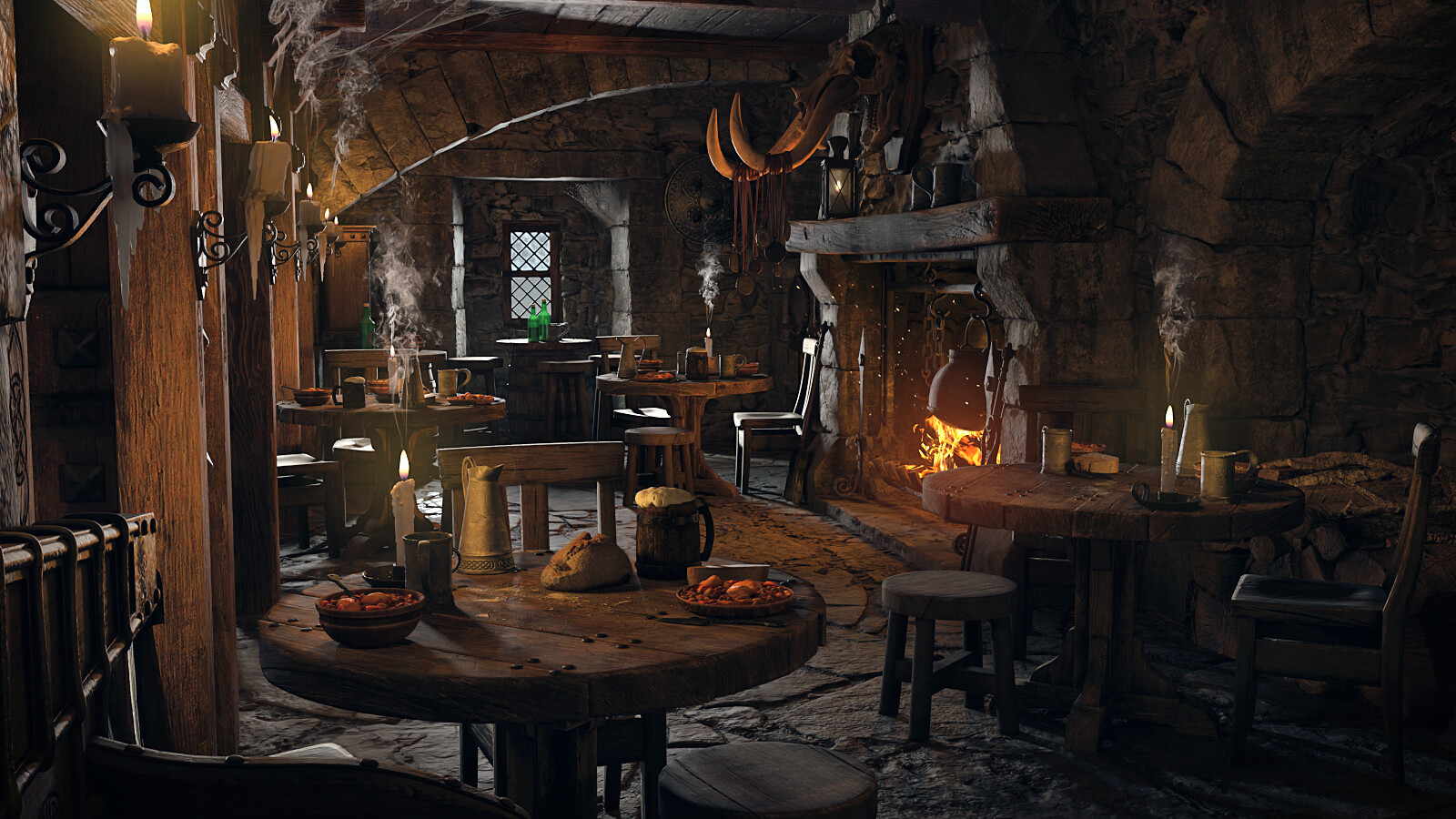This detailed illustration depicts an interior scene of a medieval pub or bar, rendered in rich browns and warm tones. Dominating the right side of the room is an ornate, large wood-burning fireplace with orange flames and sparks of light emanating from it. Above it hangs a pot suspended over the fire, a probable nod to medieval cooking styles. The fireplace, framed by an elaborate wood mantle with strong supports, also boasts a trophy sporting curved antlers.

In the bottom left of the image sits a circular wooden table, adorned with a pitcher of beer and several platters of food, surrounded by sturdy wooden chairs. Another round wooden table on the right side holds a lit white candle, its soft yellow flame providing additional illumination.

The room features towering pillars made of thick wood, and an arch below the ceiling supported by wood sections. The stone floor enhances the rustic and historical ambiance of the scene. Additionally, a window in the background, with a crisscross framework of translucent panes, allows for a peek at the exterior while contributing to the room's medieval aesthetic. This color illustration, with its apparent digital creation, evokes a fantasy setting suitable for a PC game or a richly imagined medieval narrative.